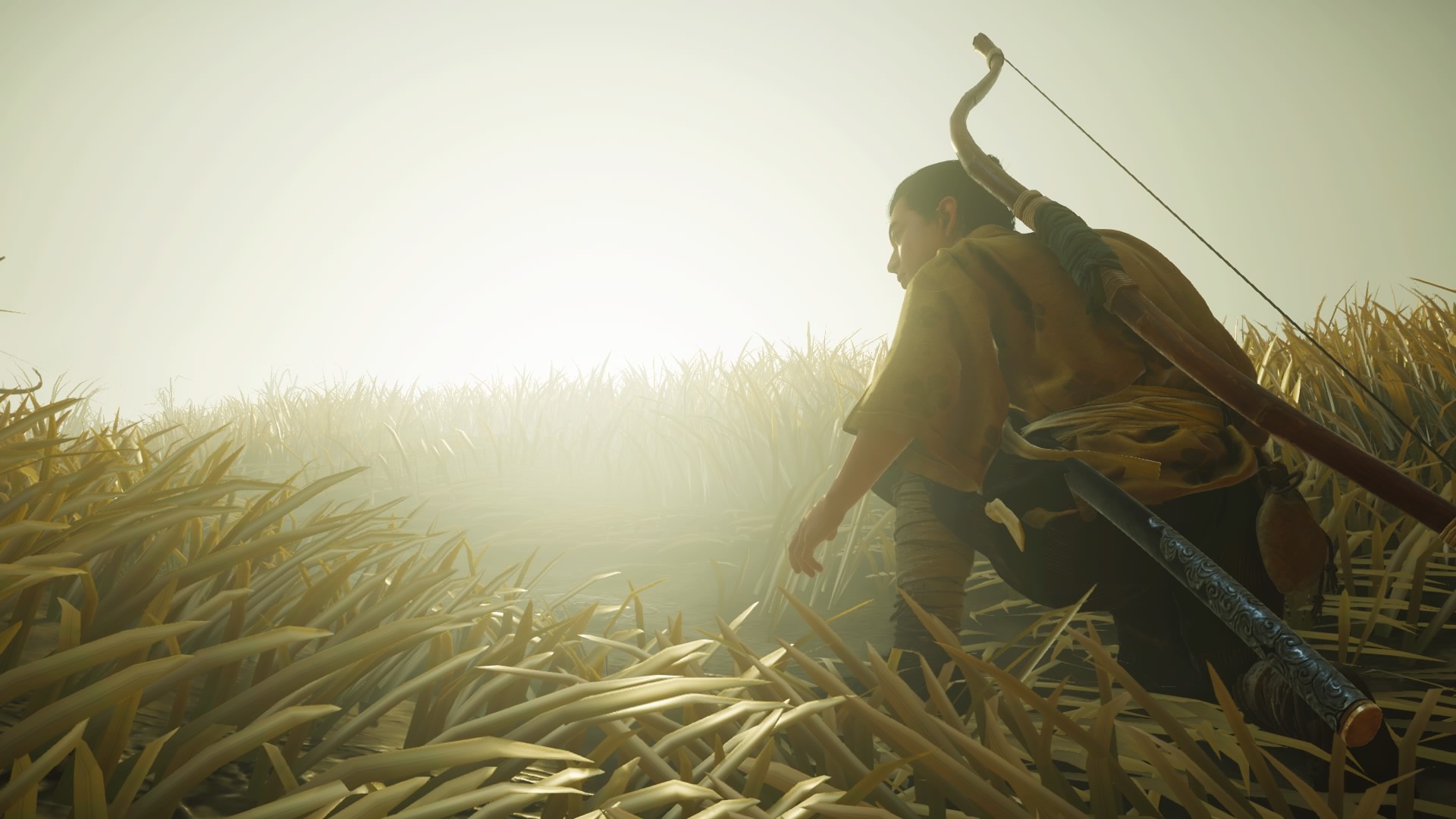In this striking, highly detailed digital art or photograph scene, an Asian man in a brown T-shirt and black pants is captured walking through a field of yellowed corn. His dark hair frames his face as he gazes off to the left. Clad in essential gear, he carries a large bow on his back, complete with a bag that features straps over his shoulders, and an ax tucked into the bag. Notably, his legs are wrapped in cloth, enhancing his rugged appearance. He navigates a path that cuts through the tall cornstalks, their top leaves barely visible against a sunlit backdrop.

The scene is dominated by the lighting of either sunrise or sunset, with a brilliant golden hue illuminating the sky. The sun, either rising or setting, casts a radiant glow across the landscape, highlighting the cornstalks and the man's profile. The cloudless sky intensifies the light's effect, enriching the atmosphere and emphasizing the serene yet purposeful moment captured in the image.